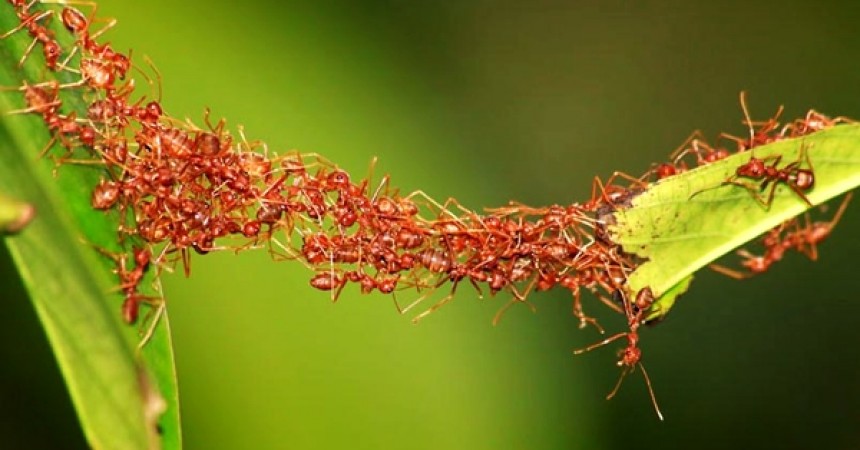This extraordinary close-up image showcases a remarkable display of teamwork among red fire ants. The ants are forming a living bridge, using their bodies to connect a smaller, dangling leaf on the right to a larger, nearly vertical leaf on the left. The background of the image is a gradient of blurred green shades, darker on the right-hand side and lighter in the middle, possibly indicating foliage. On the left bottom corner, there's a noticeably darker patch. The ants are meticulously chained together, some clinging to the left-hand leaf, others to each other, creating a sturdy bridge that spans across the middle of the image. This bridge comprises potentially over a hundred ants, making it thick enough to support additional ants, possibly for foraging or colony transport. One of the ants with a conspicuously long antenna is prominently visible, poised as if monitoring the process. This intriguing scene highlights the incredible cooperative behavior and engineering skills of these tiny insects, offering an awe-inspiring glimpse into the complexities of their world.